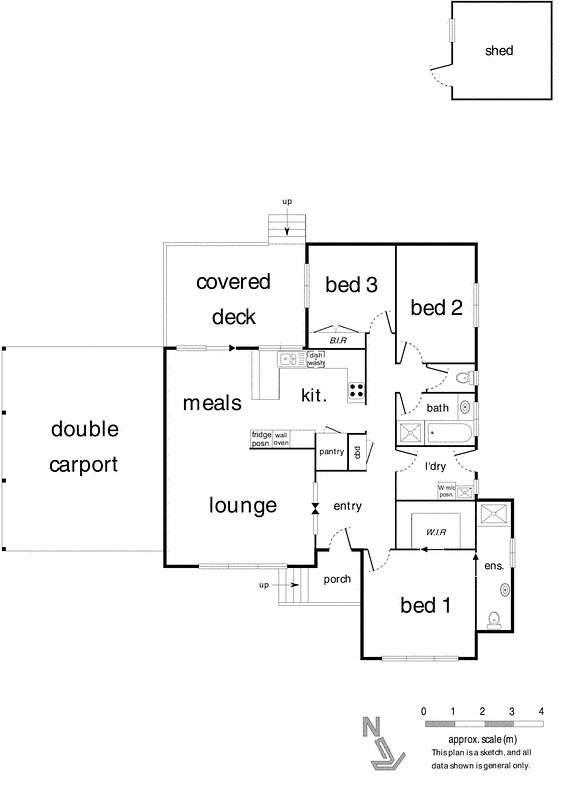This image depicts a detailed floor plan of a house, showcasing the layout of various interior rooms and features. The house is divided by numerous lines that delineate separate rooms, all clearly illuminated. Notably, there is an extension at the top right corner, distinct from the main structure, labeled "shed."

On the bottom left exterior, dotted lines form a semicircle, indicating the path of a door's swing. Central within the layout are several identifiable areas, including multiple bedrooms, a lounge, an entryway, a porch, a covered deck, a double carport, a dining area, and a kitchen. These sections are primarily separated by thick lines, with some areas demarcated by thinner lines or small empty squares.

In addition to the room designations, the bottom right of the plan features a scale bar, alternating in gray and white segments, labeled from zero on the left to four on the right, indicating the approximate scale of the drawing. This comprehensive floor plan provides a clear overview of the spatial arrangement and functional areas within the house.